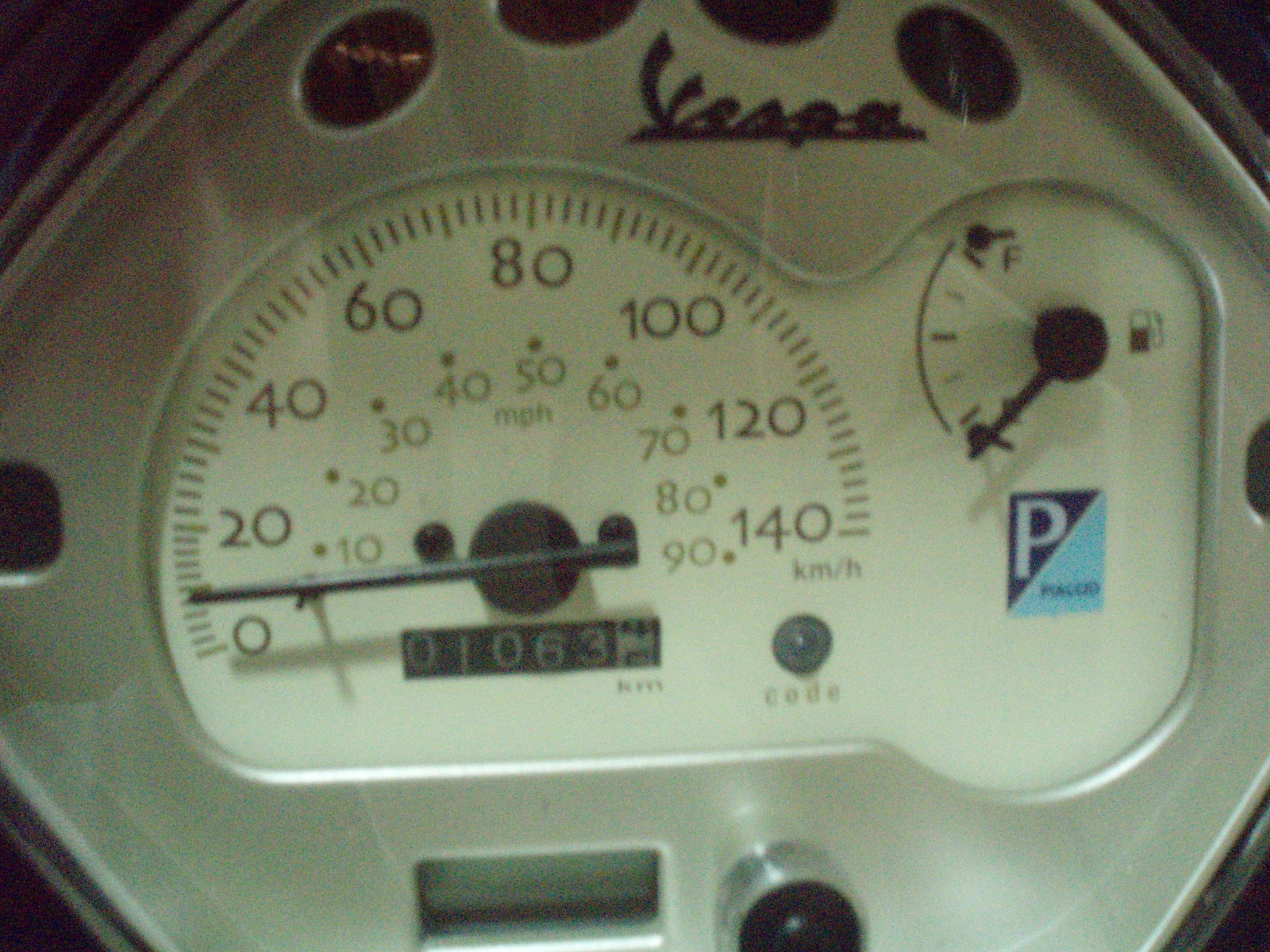Close-up of a modern Vespa scooter speedometer. The speedometer, marked in both kilometers per hour (km/h) and miles per hour (mph), displays a reading of 1,063 kilometers. The km/h scale is represented by black numerals ranging from 0 to 140, while the mph scale, denoted by dark green numerals, ranges from 10 to 90. Between the major marks, smaller lines increment by twos, with longer lines indicating tens. 

A notable feature on the panel includes a "CODE" indicator with a small switch. The scooter's parking pass, distinguished by a bright blue and dark blue triangle with a white "P" in the center, is also visible. Above the parking pass is an empty fuel gauge, suggesting the scooter is not currently running. The display shows the fuel gauge marked by a gas pump icon to the right.

The Vespa logo is prominently displayed in black letters, and four circular indicators are situated above the logo. Below the speedometer is an LED display, currently turned off, and a silver circular component with a black middle, potentially the ignition.